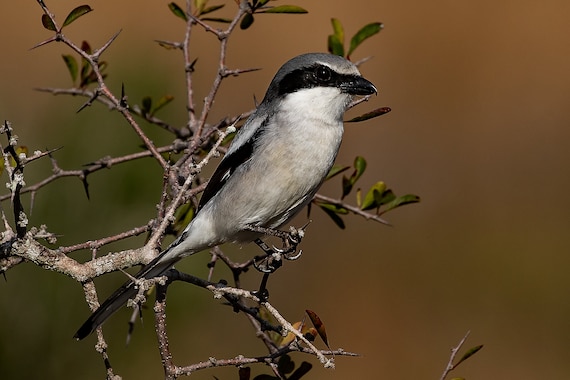The image captures a small bird perched delicately on a mostly barren, thin-branched tree. The tree is almost dead, with only a few sparse patches of leaves interspersed among the branches. The bird, centrally positioned and in sharp focus against a blurred brown and green backdrop, features a white belly, gray plumage, and distinctive black markings around its beak and eyes, giving a bandana-like appearance. Its head is partially white, complemented by a black tail and some black on its wings. The bird is gazing to the right, seemingly in search of food, providing a serene and contemplative scene.